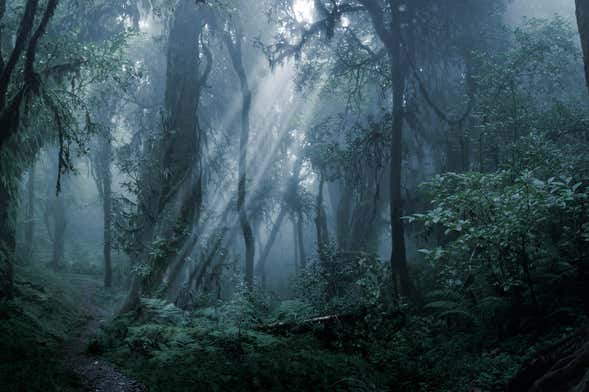This image captures a desaturated, moody scene of a dense forest, possibly resembling a rainforest like the Amazon or a northwestern forest. The photograph, likely taken during a foggy morning, has an ethereal, almost eerie atmosphere. Tall, thick trees and lush plant life dominate the scene, with mist and fog creating a veil over the forest, making it difficult to see clearly. The light struggles to pierce through the thick canopy, resulting in soft, angelic rays or "god rays" that cast a subdued, pale white light across the greenery. The colors in the image are muted, with gray-green hues blending into the shadows, imparting a sense of coldness and desolation. Despite the intricate details of the forest, it appears lifeless with no visible animals or human presence, enhancing the haunting and mysterious vibe of the photograph.